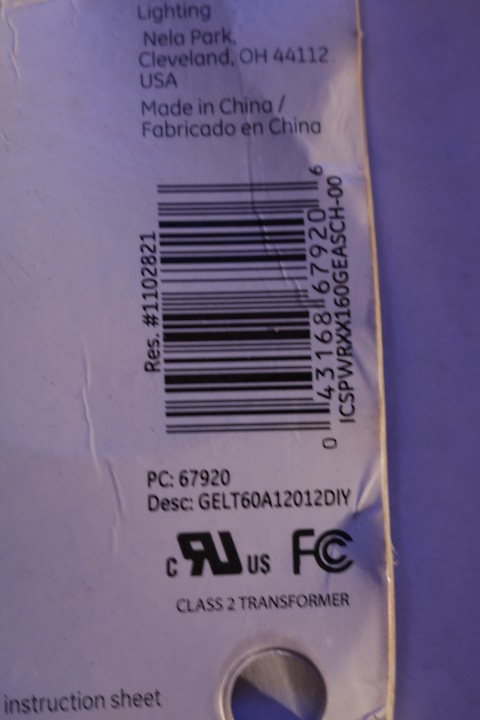The image is a detailed close-up of an informational product tag, likely for an electronic device, captured on wrinkled, beige-white paper. The text is predominantly black. At the top right, it clearly states "Neela Park, Cleveland, Ohio, 44112, USA," followed by "Made in China" and its Spanish translation, "Fabricado en China." Below these details is a vertically oriented barcode with the number PC67920. The bottom part of the tag features the designation "Class 2 Transformer" and the words "Instruction Sheet" on the bottom left. Additionally, there is a conspicuous round hole punched out at the bottom right, possibly for hanging the tag. The tag also includes various logos like FCC certifications and may appear to have more product numbers or codes. The overall impression is that of a comprehensive label providing essential manufacturing and product information.